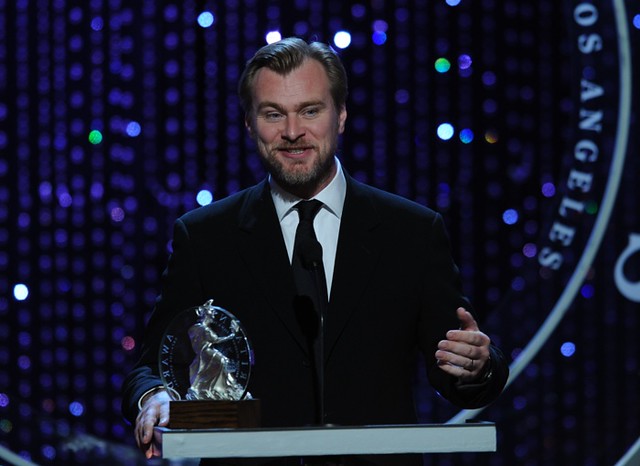The image captures an award ceremony set against a backdrop of multicolored lights—blue, green, white, and more. Front and center is a man in a black suit, white shirt, and black tie. He stands behind a dais, gripping it with his right hand while his left hand makes animated gestures. The man, who has neatly combed hair and facial hair, is smiling at the audience. The dais features a microphone with a white border and an award or trophy. The trophy, resting on a wooden brown base, includes a statue of a lady and a glass circle bearing some text. Although the text and logo on both the background screen and the trophy are not fully visible, "Los Angeles" is discernible. The overall atmosphere suggests a formal and celebratory event.